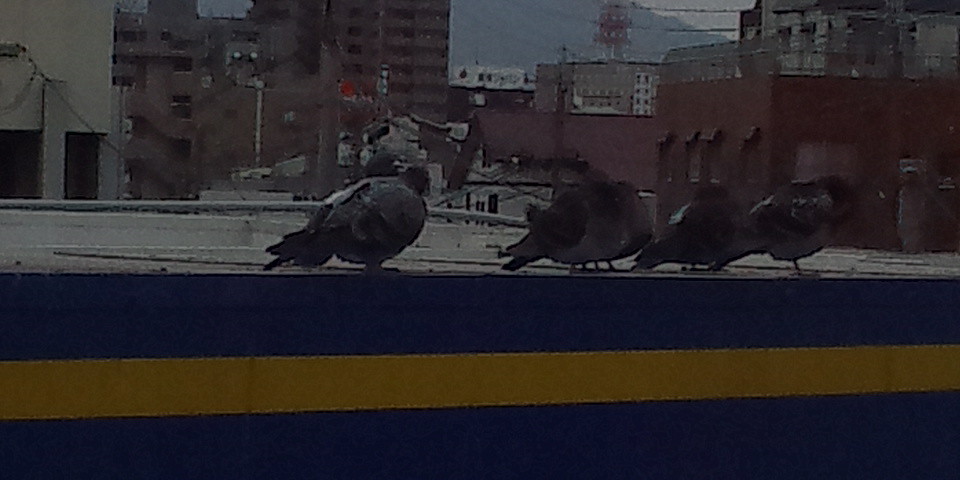In this dark, low-quality outdoor photograph, an evening city skyline forms the backdrop, featuring a mix of tall brick and concrete buildings, light poles, and distant mountain slopes under a gray sky. Dominating the middle of the image is a large brick building, while in the foreground, a flat rooftop with a blue top and a horizontal yellow stripe comes into view. Along the edge of this roof, four gray pigeons, also known as rock doves, are lined up in a horizontal row, mostly facing to the right with their tails to the left. Three of these pigeons appear to be pecking at something atop the roof, while they all gaze over the town below, seemingly observing the evening activities.